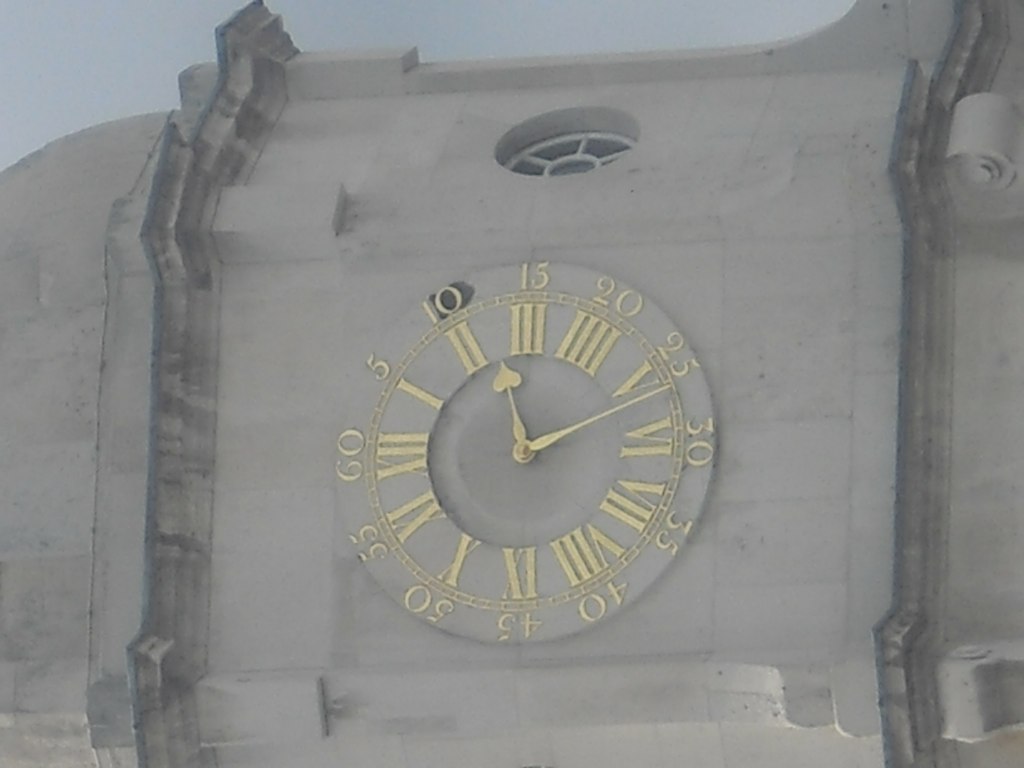In this image, a large, imposing concrete building dominates the scene. On the left side of the structure, massive concrete blocks appear to form a series of steps ascending to the top. To the right, several external units, possibly air conditioning systems, are mounted along the building's facade. Centrally located on the vast expanse of concrete is a distinct circular feature—a window with multiple panes arranged in a floral pattern. Above this intricate window, a monumental concrete clock is displayed, its face adorned with gold Roman numerals. The clock's hands also feature gold detailing, with the minute hand uniquely marked by a spade design, while the hour hand remains long and slender.